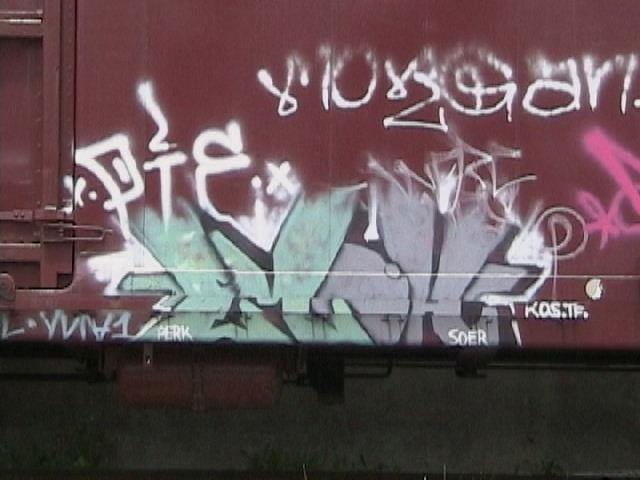This detailed close-up photograph captures a section of a red, rusty train compartment, prominently featuring a metallic red valve. The valve is adorned with vibrant graffiti, incorporating white, light blue, purple, and pink colors. The graffiti includes elaborate and colorful letters, with notable text such as "PERC" in large white capital letters and "SOER" further to the right, also capitalized. Above "PERC," "P-T-E" is written prominently, with green symbols resembling an upside-down 7 and a Y nearby. Additionally, the letters O and H are rendered in gray with black outlines, giving them a 3D appearance and flame-like details. More graffiti, including "RO.SITF." and "81082 at ARL" can be seen above, all set against the red expanse of the train side. At the bottom of the image, a gap reveals a portion of the gray background wall and some grass. Latches for opening the cargo area are visible to the left of the composition, emphasizing the industrial and worn nature of the train compartment.